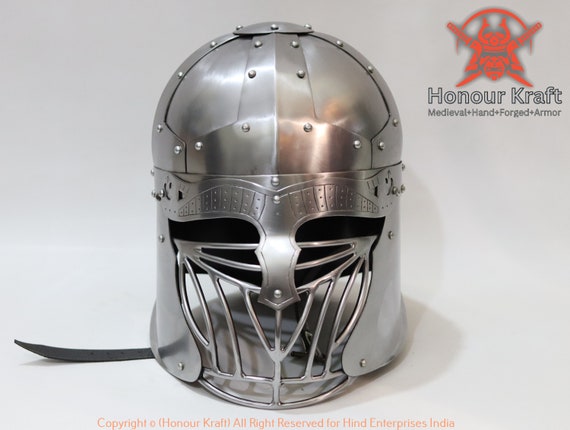This indoor photographic image features a modern, custom-made medieval-style helmet positioned centrally. The helmet boasts a polished, silver-colored dome that provides full protection for the top of the head. Along its sides are ear guards, while the front area has an eye opening shielded by a mask, ensuring visibility and safety for the wearer. The nose is protected by a solid central piece, with thin bars below safeguarding the mouth area. The helmet is adorned with small knobs throughout its surface, adding to its intricate design. To the left of the helmet, a strap is visible. In the top right corner, an orange graphic depicts a warrior's head with horns, helmet, and two crossed samurai swords. Adjacent to this logo, text reads "Honorcraft Medieval Hand Forged Armor." At the bottom of the image, additional text states "copyright Honorcraft All Rights Reserved for HIND Enterprises India."